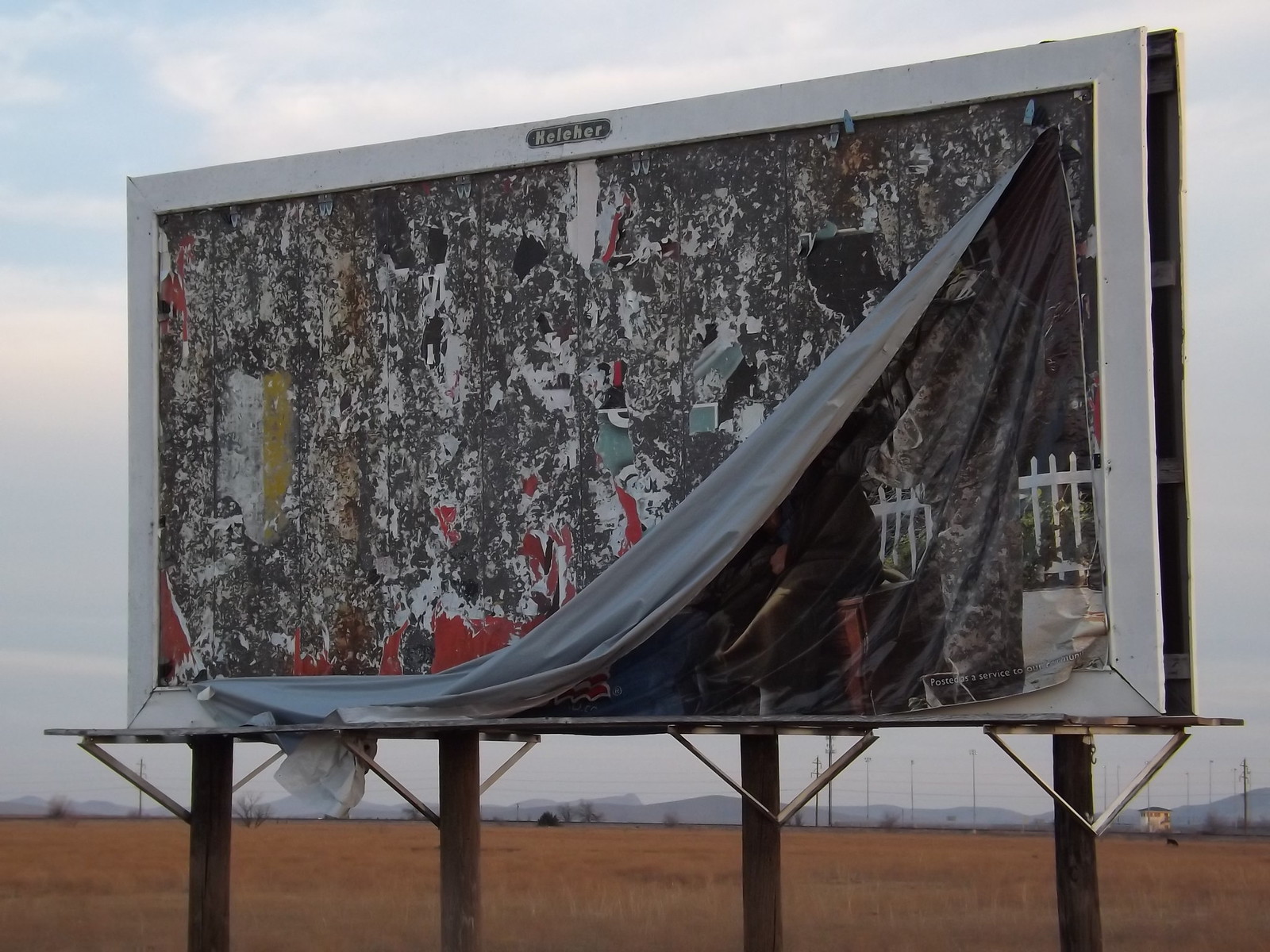The image depicts a close-up of a deteriorating billboard standing along a highway, approximately 10 feet off the ground, supported by four wooden telephone poles. The billboard is in a flat, grassy or dried-out pasture area with a backdrop of utility poles, cloudy skies, and distant mountain ranges. The billboard's white frame is marred by patches of grey, white, red, and black remnants of previous advertisements. A large cloth advertisement, once affixed to the billboard, is in the process of falling apart. It remains attached only at the upper and lower right-hand corners, while the rest of the fabric hangs loosely, obscuring the original content, which shows a tree and a white picket fence. The scene is cast in dim lighting, enhancing the sense of abandonment and decay.